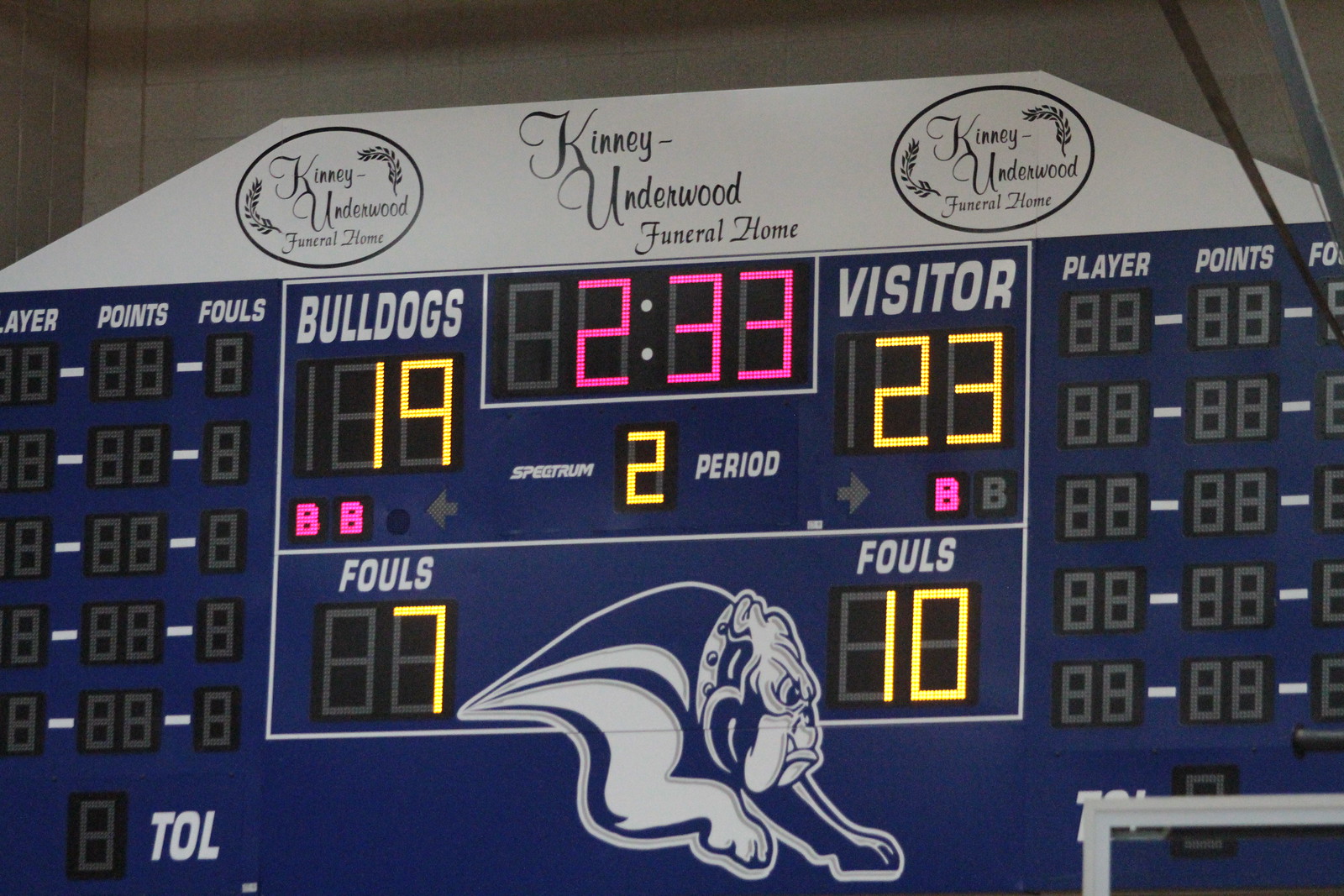The photograph showcases a detailed view of an indoor scoreboard, predominantly in dark blue with contrasting white writing. The scores, displayed in bright yellow-neon colors, show "Bulldogs" with 19 points and "Visitor" with 23 points. The timer is highlighted in a striking neon pink. Notably, the scoreboard is sponsored by Kinney Underwood Funeral Home, with the name prominently displayed three times: once in the center at the top and within ovals on both the left and right sides. The font used for the sponsor's name is slightly italicized, adding a touch of elegance.

At the bottom center of the scoreboard, there is an illustration of a fierce, action-ready white bulldog, symbolizing the home team. The scoreboard is comprehensive, including information on fouls, with the Bulldogs having seven and the Visitors having ten. The overall layout effectively delineates the home and visiting teams' data, presenting a clear and detailed visual representation of the ongoing game.